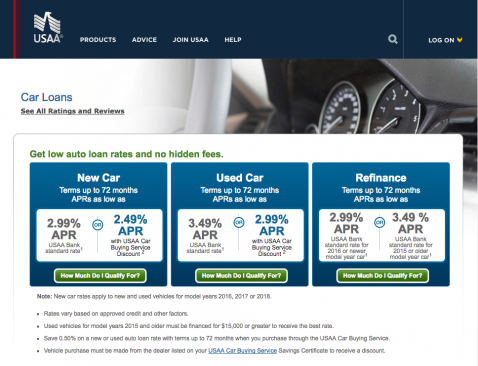The webpage for USAA features a sleek, black header adorned with the USAA logo in white. It includes navigation options: "Products," "Advice," "Join USAA," and "Help," all rendered in white text. Adjacent to these options is a white magnifying glass icon for search functionality and a "Logon" button in white text, accompanied by a yellow drop-down arrow.

Below the header, the main section of the page showcases an image of a vehicle's interior. Overlaid on this image, "Car Loans" appears in blue text, with "See All Ratings and Reviews" in black text beneath it. The interior depiction highlights a steering wheel, along with a speedometer and tachometer on the car's instrument panel.

Further down, there is a prominent rectangular section with a white background. It features the message "Get low auto loan rates and no hidden fees" in green text. The section is divided into three distinct squares, each detailing different loan options:

1. **New Car**: Terms up to 72 months with APRs as low as 2.99% or 2.49%. 

2. **Used Car**: Terms up to 72 months with APRs as low as 3.49% or 2.99%.

3. **Refinance**: Terms up to 72 months with APRs as low as 2.99% or 3.49%.

Each square includes small, black text beneath the APR rates, which is difficult to read, and a green button labeled "How much do I qualify for?" at the bottom.

Finally, there are five additional lines of small black text that are hard to decipher, positioned immediately following the loan details.